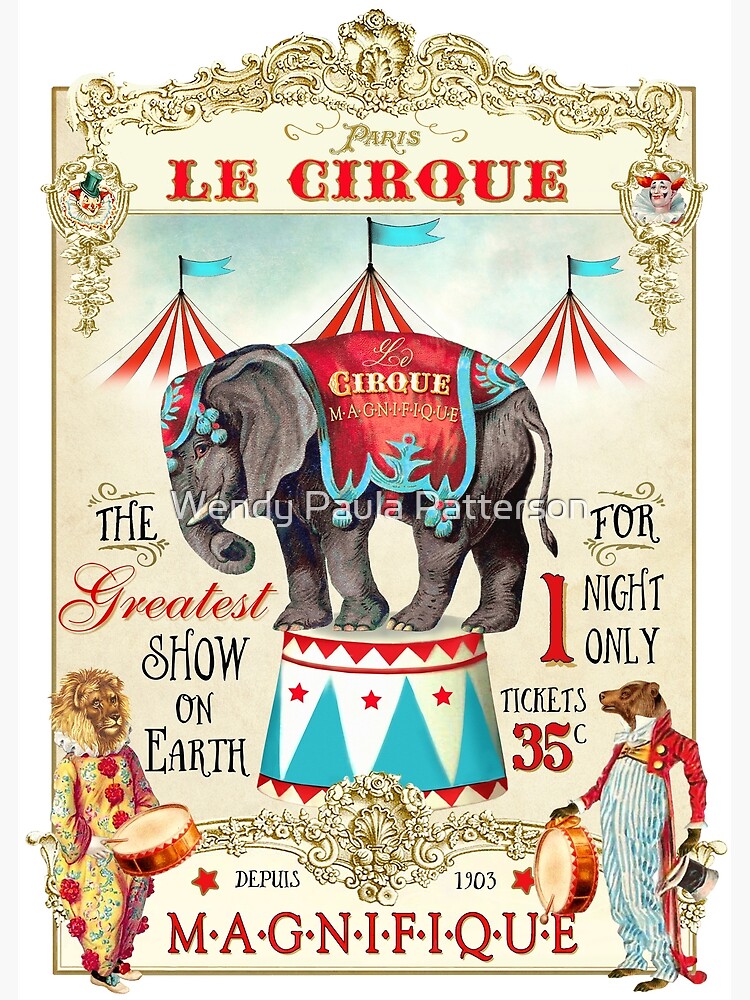This vintage 1903 circus poster, featuring a rich, golden-bordered portrait orientation, intricately designed with hand-drawn ornate, floral patterns along the top and sides, advertises "Les Cirques" in Paris. The once white background has aged to a beige hue, accentuating the classic look of the design. Central to the poster is a majestic elephant adorned with turquoise and red attire, standing proudly on a red, blue, and white pedestal. Behind the elephant, colorful circus tents with red, white, and blue stripes and blue flags are visible. To the left, a lion dressed in a clown outfit with red buttons and funny shoes plays a drum, while to the right, another figure, possibly a bear in a ringmaster outfit with a short red jacket and golden buttons, also plays a drum. The poster touts itself as "The Greatest Show on Earth," with tickets priced at 35 cents for a one-night-only performance. The French phrase "Magnifique" is prominently displayed, emphasizing the grandeur of the event, alongside the watermark "Wendy Paula Patterson" in the center. The top of the poster also features scrollwork designs and images of a clown and possibly an acrobat, further emphasizing the festive and artistic nature of this timeless advertisement.